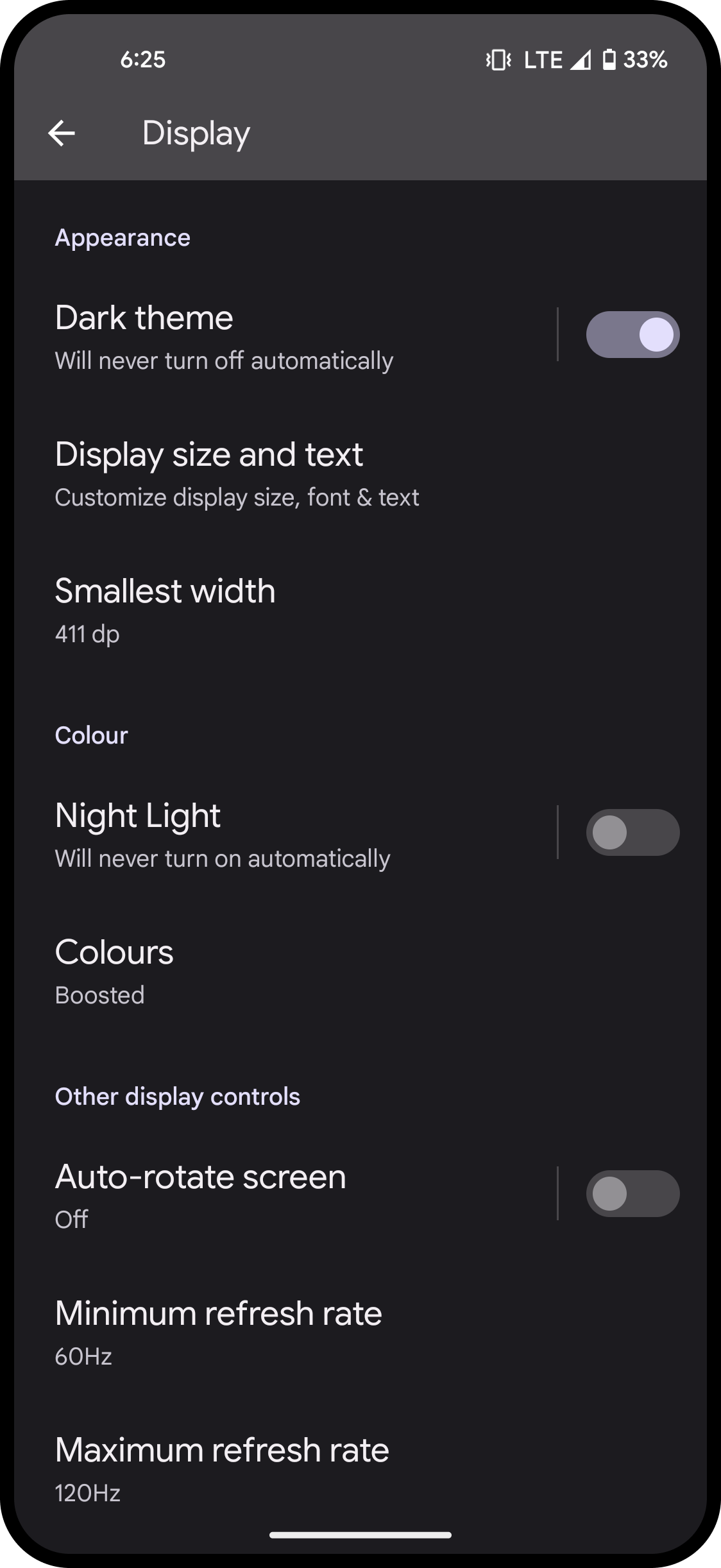This mobile screenshot features the display settings menu, captured against a black background. At the very top, there's a dark grey status bar displaying the time as 6:25, alongside icons indicating vibrate mode, LTE connectivity, cellular signal strength, and a battery level at 33%. Below this, a navigation bar with a right-facing arrow, a left-facing arrow, and the label "Display" in white text is present.

The primary content of the screenshot is organized into three main sections within the display settings menu:

**1. Appearance:**
   - **Dark Theme:** Not toggled on.
   - **Display Size and Text:** Includes an option for adjusting the smallest width.

**2. Color:**
   - **Night Light:** Not toggled on.
   - **Colors:** Set to "Boosted" mode.

**3. Display Controls:**
   - **Auto-Rotate Screen:** Disabled (toggled off).
   - **Minimum Refresh Rate:** Set at 60Hz.
   - **Maximum Refresh Rate:** Set at 120Hz.

Each section is organized in a clear, concise manner, allowing the user to easily customize their display settings.